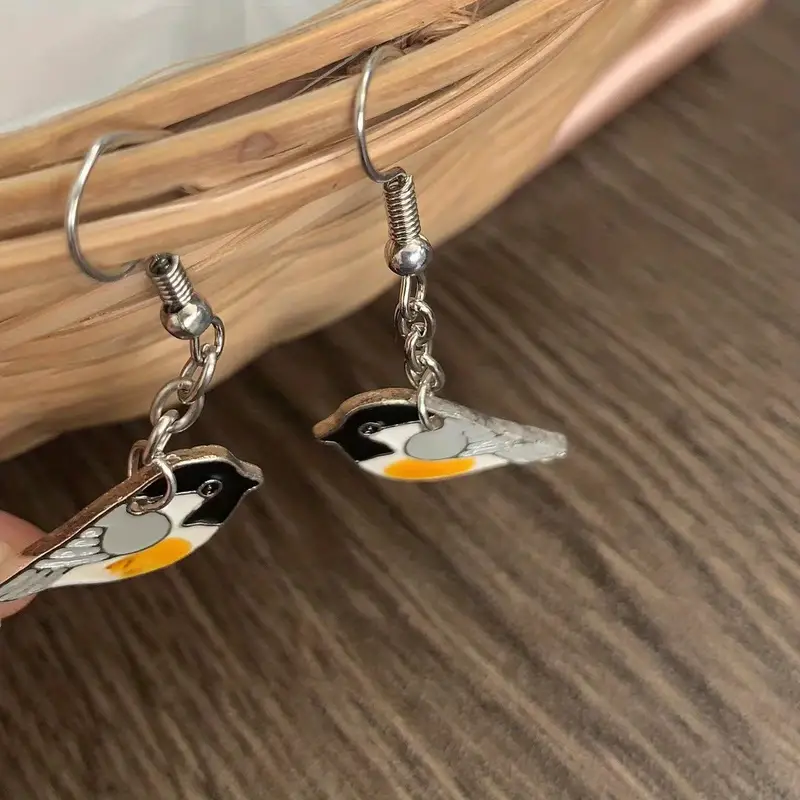This image is a highly detailed close-up shot of a pair of bird-themed earrings. The earrings, crafted from what appears to be sterling silver, feature detailed small birds with a striking color palette: black heads, white cheek areas, gray wings, and orange bellies. The birds are positioned to face each other, highlighting their intricate design. The earrings are suspended by silver hooks onto a tan, possibly wicker, object. This base, though partially visible, appears to be placed on a surface that features streaks of different shades of brown, giving a textured backdrop. A small, flesh-colored area to the left suggests a human hand might be part of the composition, likely holding one of the earrings. Overall, this image serves as an elaborate product shot, portraying the earrings in a visually appealing manner.